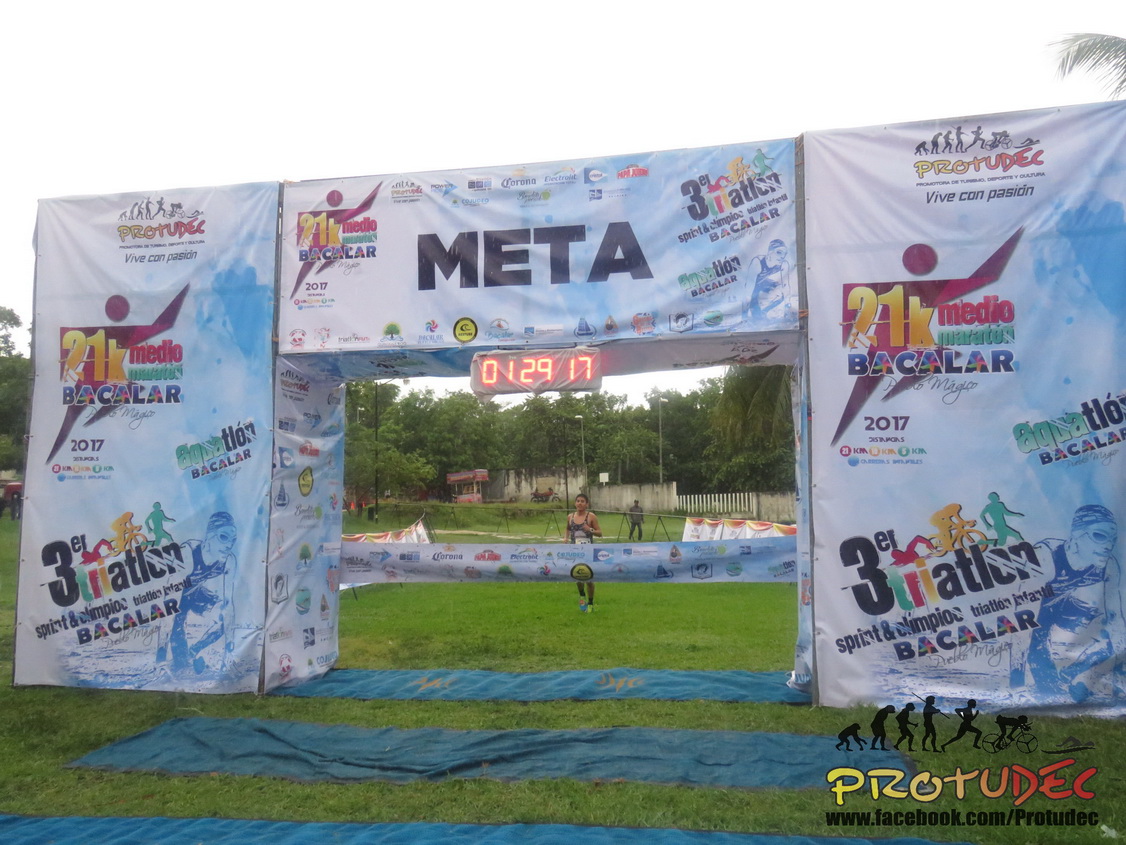In this vibrant outdoor setting, a grassy field serves as the stage for the climactic moment of a race. At the foreground, a solitary runner is about to cross the finish line, marked by a prominent banner extending horizontally across the frame. The archway above the finish line bears the word "META" in bold black letters, with additional text and logos indicating a 21K race, as well as the year 2017. The logo features a caricature of a runner with an arm extended upward.

Surrounding the finish area, blue rubber mats lie on the grass, flanked by barriers adorned with various advertisements. Among these ads, a Facebook logo "Pro2Deck" and a visual progression from monkey to man are notable. To the right of the finish line, there's a man who appears to be a photographer, standing near a white picket fence. Behind the fence, trees frame the scene under a pale sky, further suggesting the race is taking place in broad daylight.

The array of colors—greens of the grass, blues of the mats and sky, and various hues from the runners' attire—create a dynamic and lively atmosphere.